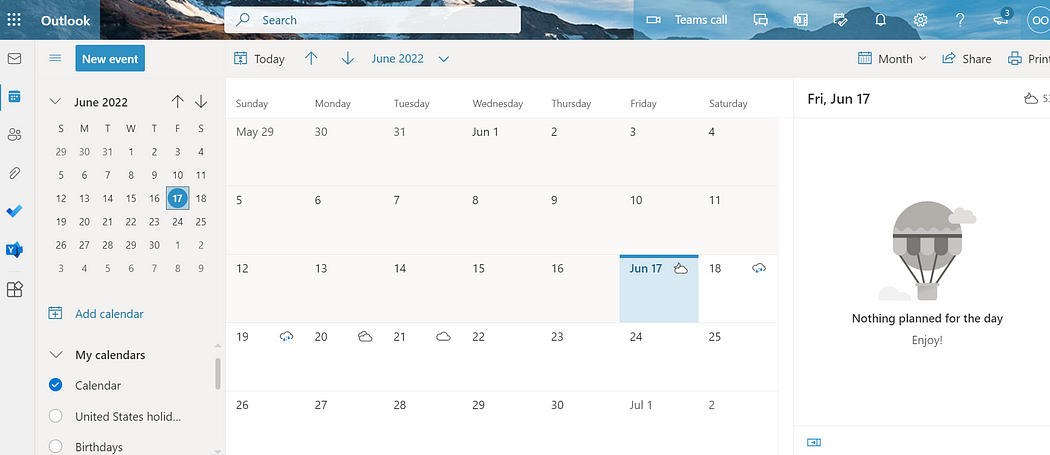The image displays a Microsoft Outlook calendar interface, showcasing organizational and navigational elements in a highly detailed manner. The interface features a prominent blue banner at the top, adorned with a subtle mountain range graphic in the background. In the upper left-hand corner, the word "Outlook" is displayed, adjacent to a search bar emblazoned with the prompt "Search."

On the upper right-hand corner, a suite of icons is visible, including a video button for initiating team calls, followed by icons for messages, notifications, settings, help, and an intriguing telescope symbol marked with a number three, the latter's function remaining ambiguous. Further along, options for creating a "New Event" are available.

The calendar is set to June 2022, with Friday, June 17th specifically highlighted, indicating no scheduled plans for the day and encouraging the user to enjoy their free time. The calendar grid organizes days of the week in a standard layout from Sunday to Saturday, spanning dates from May 29th to July 2nd.

On the sidebar, options include "Add Calendar" and "My Calendar," with "Calendar" selected by default, while "United States holidays" and "birthdays" remain unchecked. Additionally, the far left-hand side houses further options for attachments and other utilities, though these remain unused in the current view.